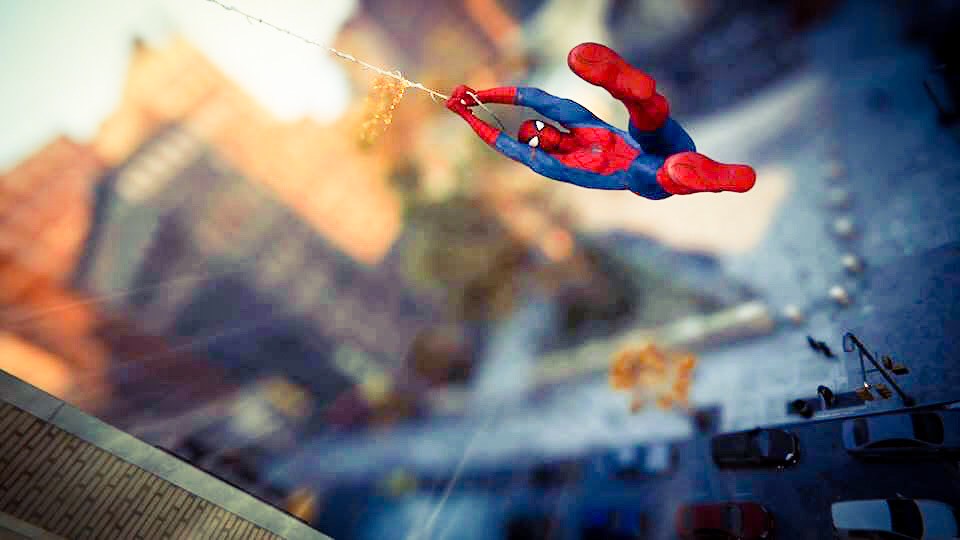In this ultra-realistic 3D image bursting with vibrant colors, Spider-Man is dynamically captured swinging on a thick web around the corner of a towering, brownish-red brick building. Positioned towards the top right of the frame, Spider-Man's iconic red and blue suit, complete with black webbing details and striking white eyes, stands out dramatically against the blurred cityscape behind him. With both hands firmly grasping his web, he appears in mid-swing towards the viewer, giving a thrilling sense of motion. 

Below, a bustling street filled with around ten cars adds a sense of urban energy and depth. The perspective suggests a dramatic angle, as if the shot was captured while he was in the midst of a daring maneuver around the building's edge. In the center of the cityscape, a vague outline of a cement park area, possibly with a tree, can be discerned, although the rapid motion blur obscures exact details. The entire scene evokes the excitement and dynamism characteristic of Spider-Man's high-flying adventures.